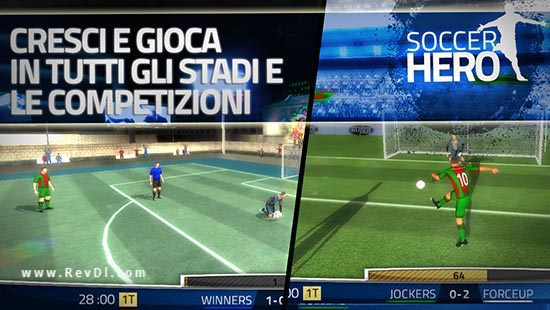This composite image is captured from a soccer video game and is divided into two distinct sections.

On the left side, the screen is in Italian, featuring a semi-crude drawing of three soccer players on a field. Despite the basic, non-realistic artistic style, the scene vividly depicts an opponent having just kicked the ball into the net, with the goalie seen on his knees in an apparent attempt to block the shot. The text reads '28 seconds, 1T,' indicating the time and possibly the period of the match, with the score showing 'winners, 1-0.' Additionally, the bottom of this section includes the URL 'www.revdi.com' in white letters.

The right side displays a screenshot labeled "Soccer Hero," showcasing a more realistic in-game scenario where a soccer player is captured in mid-action, kicking the ball towards the goal. The ball is visibly in motion, and the goalie stands alert in the net. A player's shadow can be seen on the left side, suggesting another player is out of frame. The green field adds a vibrant background to the scene. The text at the bottom shows '001T, jockers, 0-2,' indicating the teams and their scores, with the phrase 'force up' included.

Together, these contrasting images provide a detailed look into the immersive and varied aesthetics of the soccer video game, highlighting both artistic and realistic elements of gameplay.